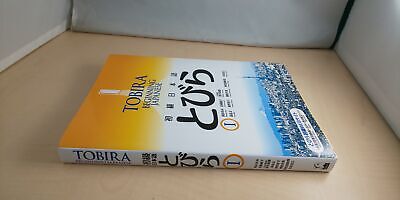The image depicts a paperback book lying flat on a light tan surface, likely the bottom of a white box, with three white sides visible around it, giving the impression of a container. The book appears to be a Japanese textbook titled "Tobira," as indicated in both English and Hiragana on the cover. The cover design features three distinct sections: the top section is yellow with a sunset streak and possibly a tower silhouette; the middle section is white with black text and Hiragana characters; and the bottom section depicts a bluish Tokyo skyline, including notable landmarks such as the Tokyo Tower and Mount Fuji. The spine of the book also prominently displays the word "Tobira" at the top, along with additional Japanese characters. A yellow circle, which might be part of the publisher's logo, is present in the middle of the cover and on the spine. This detailed scene clearly suggests that the book is used for learning Japanese.